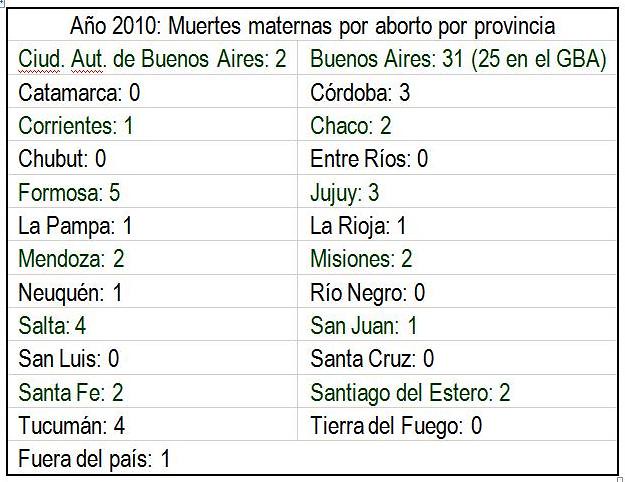In this rectangular image, we see a detailed table of information written in Spanish, printed in black on a white background. The heading reads, "Año 2010, muertes maternas por aborto por provincia," indicating maternal deaths due to abortion by province in the year 2010. The table is organized into two main columns, each listing province names alongside corresponding numbers.

The most prominent place name is Buenos Aires, with a notably high number of 31. Other locations listed include Catamarca with 0, Córdoba with 3, Fuera del País with 1, and Tierra del Fuego with 0. Most of the numbers associated with the provinces are small, typically in the range of 0 to 3, highlighting the relative frequency of occurrences. The simplicity of the table allows for a clear comparison between the different provinces, although the exact significance of the numbers requires additional contextual knowledge of Spanish.